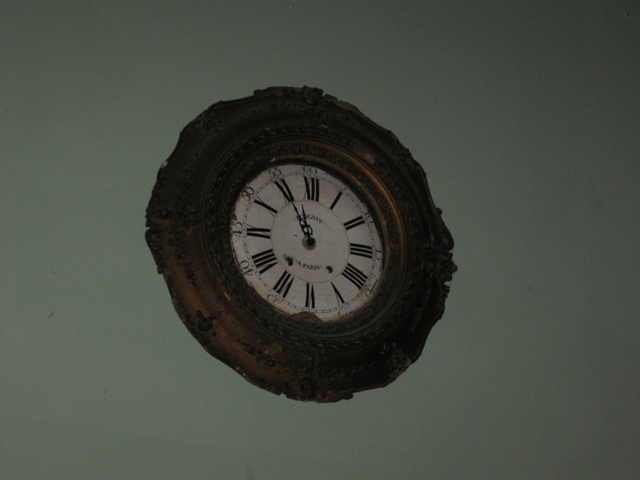This image is a color photograph of a wall clock hanging on a plain gray, or possibly gray-green, slate-colored wall. The clock's most striking feature is its thick, ornate wooden frame, which is richly carved and embossed, suggesting an antique quality. The frame is a dark, reddish wood with fluted edges and intricate floral designs. The face of the clock is white and encircled by a thin gold metal band. Roman numerals marking the hours are prominently displayed in black, with Arabic numerals above them indicating minutes in intervals of five: 5, 10, 15, and so on up to 60 at the top. The clock's black hands, one for hours and one for minutes, point to the time, which is five minutes to twelve. Although there's some illegible wording on the clock face, the overall appearance is classic and elegant, highlighting the craftsmanship of its design.